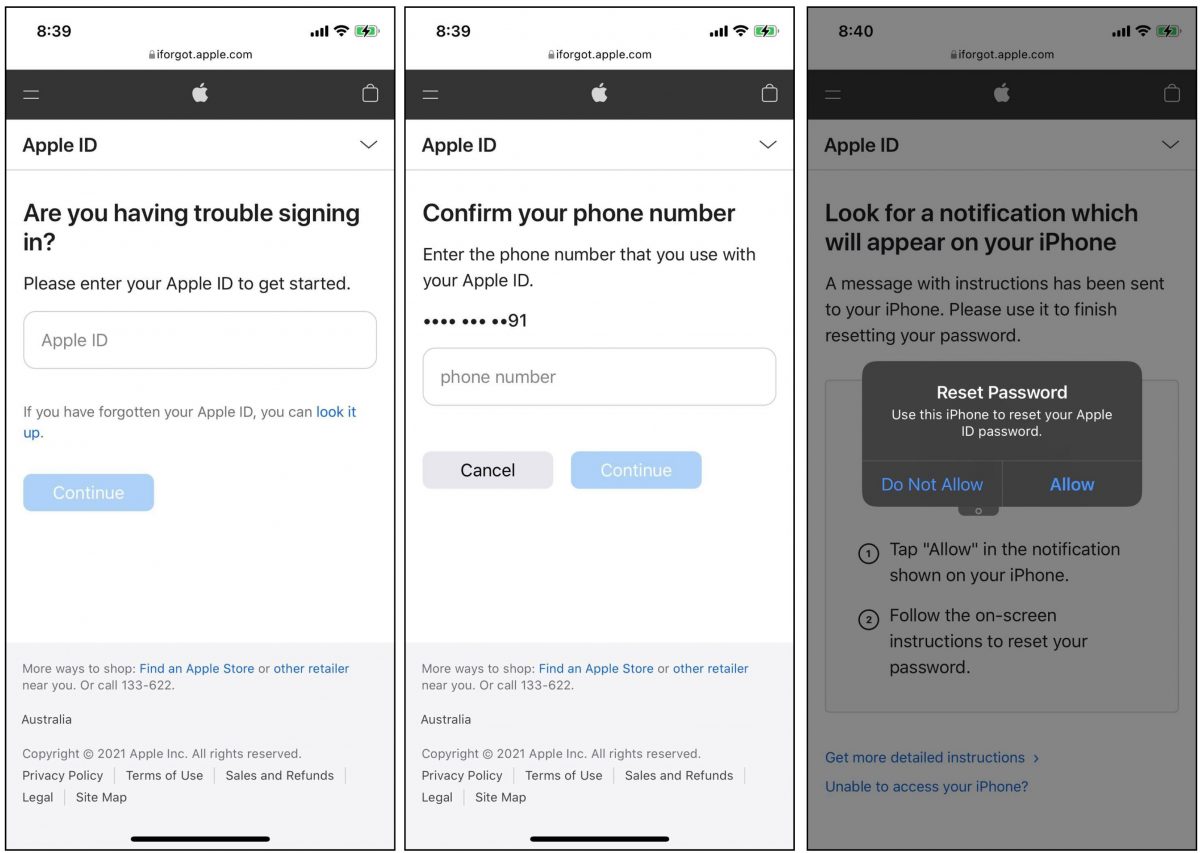The image is a diagram consisting of three side-by-side mobile phone screenshots that illustrate a sequence of troubleshooting instructions for resetting an Apple ID password. The first screenshot, positioned on the left, displays the Apple ID interface with a prompt at the top asking, "Are you having trouble signing in? Please enter your Apple ID to get started." The middle screenshot shows the next step, where the user is asked to confirm their phone number associated with their Apple ID. The phone number is partially obfuscated, revealing only the last two digits, "91." The final screenshot on the right features a grayed-out background with a dark gray window displaying the message, "Reset Password. Use this iPhone to reset your Apple ID password." Below this message are two clickable options in blue text: "Do Not Allow" on the left and "Allow" on the right. This final panel completes the process for users to reset their Apple ID password if they have forgotten it.